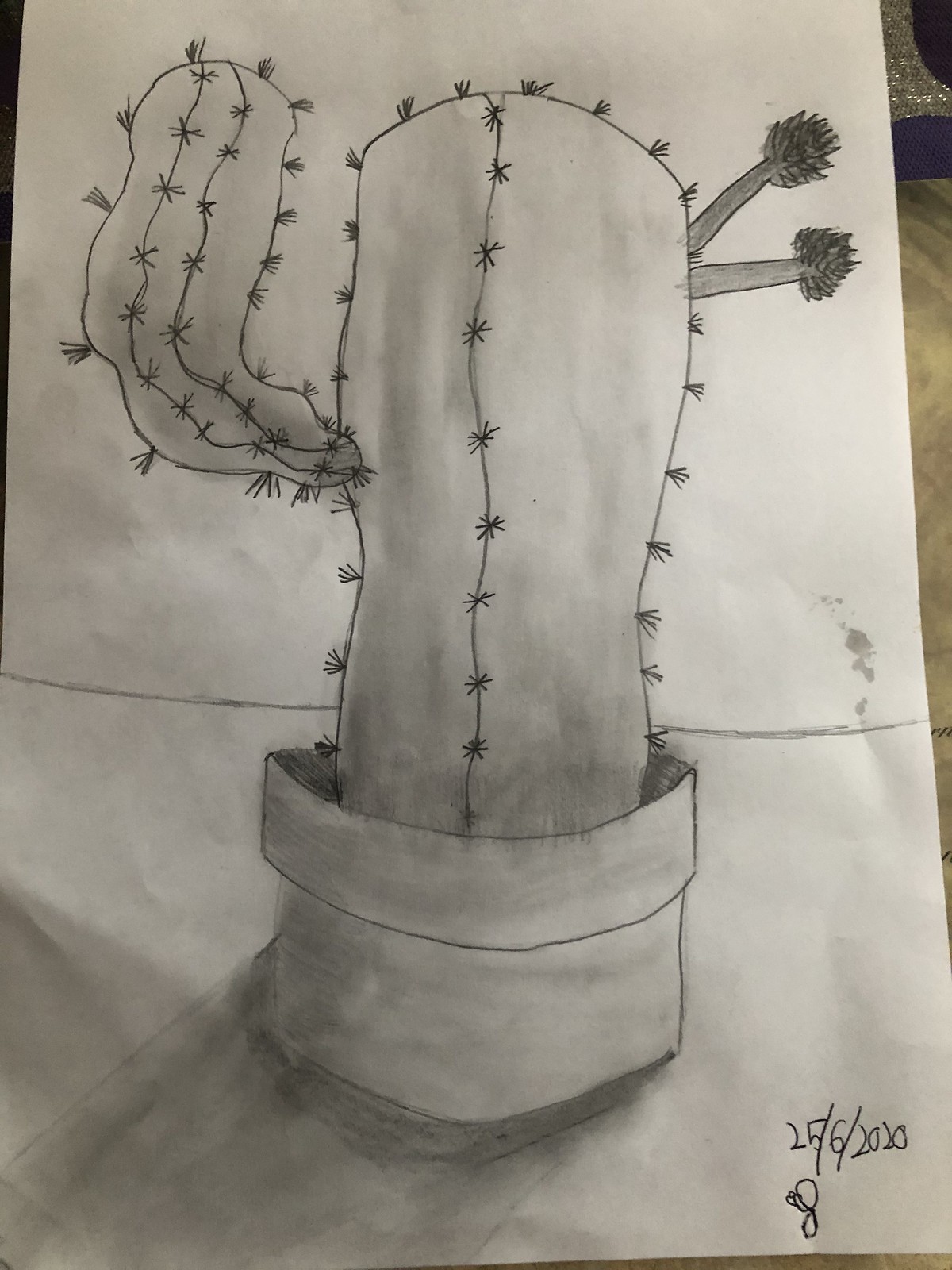A meticulously detailed pencil drawing on crisp white sketch paper features a tall cactus in a pot. The cactus, adorned with rows of tiny, sharp spines, exhibits character with an "elbow joint" arm protruding from its left side. From the top right, two small branches extend, each capped with delicate flowers adding a touch of elegance to the resilient plant. The pot, appearing modest and close to the ground, casts a subtle shadow stretching towards the bottom left corner, adding depth and dimension to the artwork.